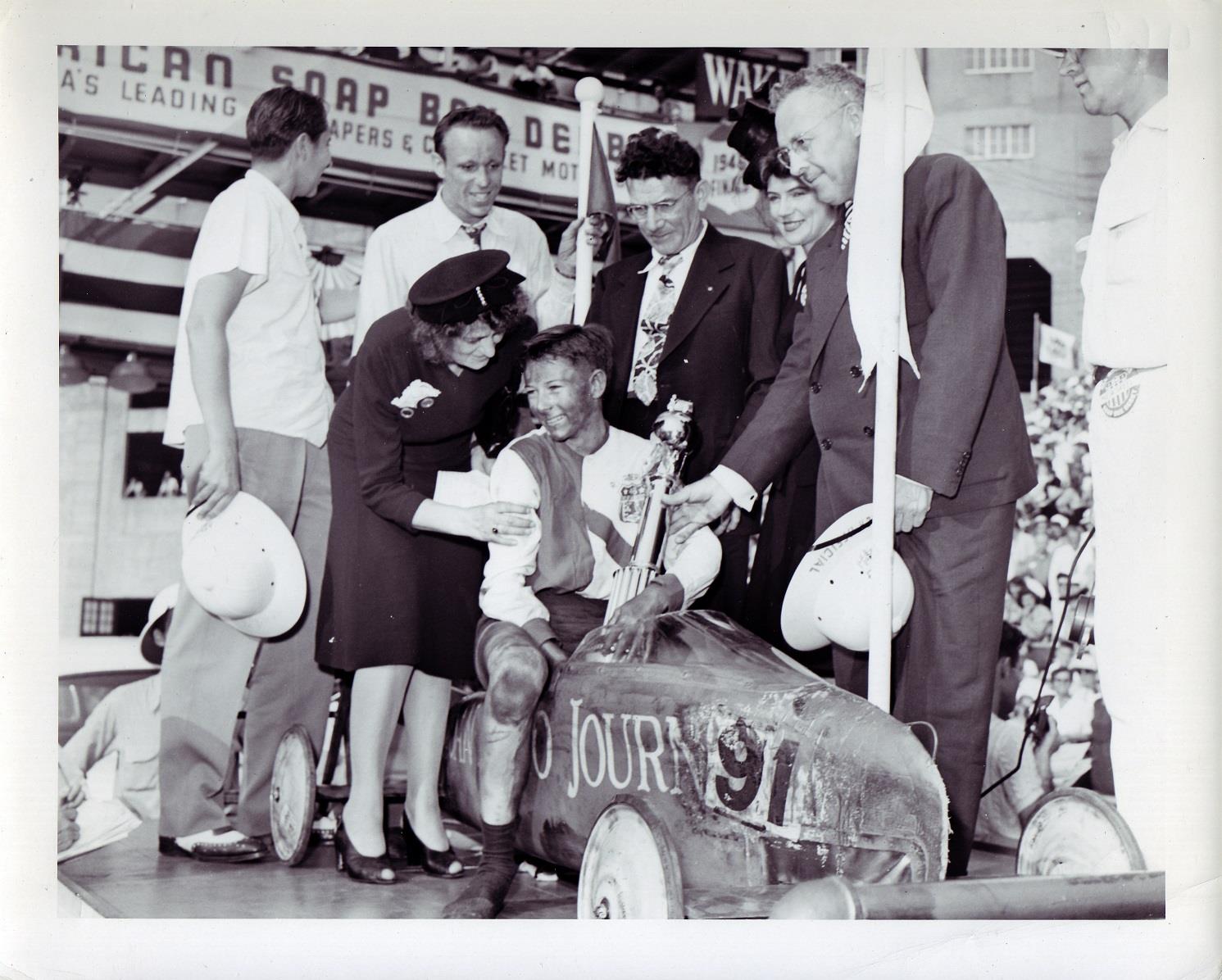This detailed black and white photograph captures the celebratory moment at a Soapbox Derby competition. At the center of the image, a young boy, around 13 years old, with a dirty face and arms likely from working on his car, sits proudly in a wooden derby car marked with the number 91. He's wearing a white shirt and holding a tall trophy in his left hand. Standing behind him, a woman in a long black dress and hat lovingly places her left arm on his back while grasping his right arm with her right hand. Surrounding them, several adults, mostly dressed in suits, are visibly congratulating the boy. One man in a suit and glasses is handing the trophy to the boy, while another man dressed entirely in white, partially visible, watches the scene. In the background, a white banner with the words "Soapbox Derby" hangs, marking the occasion as a notable event. Some officials, identifiable by their pith helmets labeled "official", add a sense of formality and importance to the scene. The image beautifully captures a moment of triumph and community in this classic racing competition.